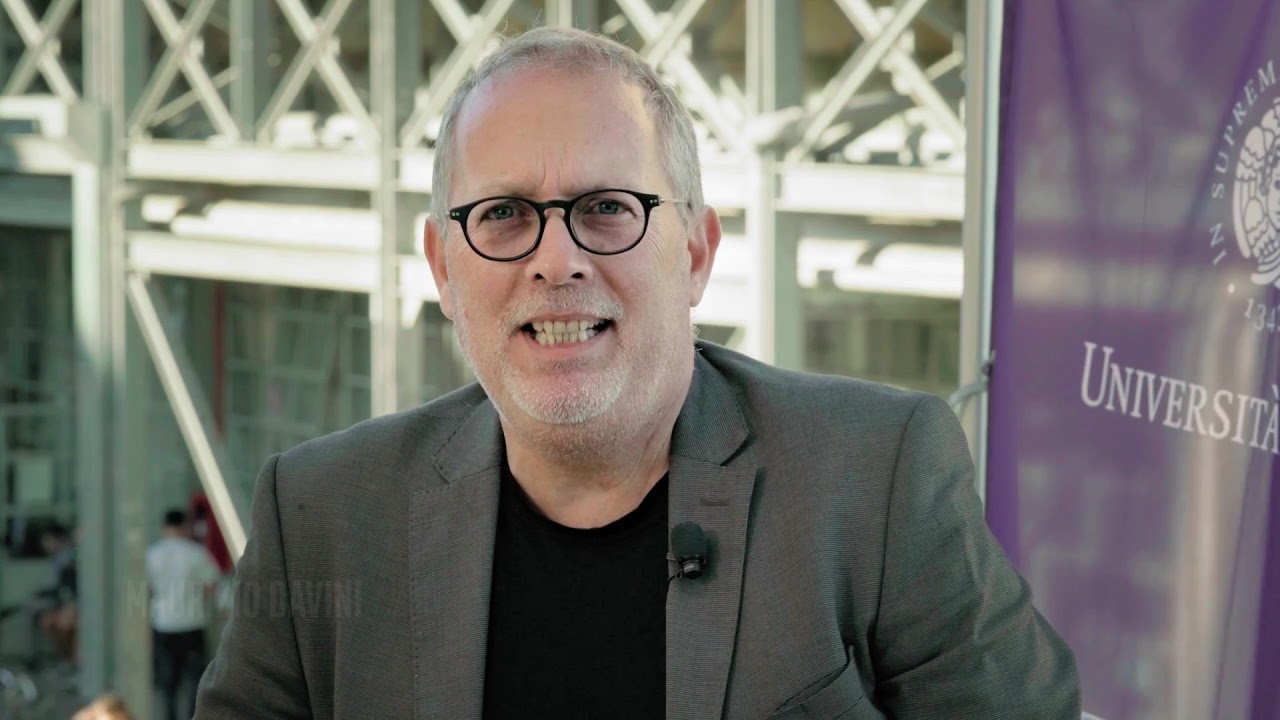The image depicts an older Caucasian man with short, graying hair that is slightly balding and a white and gray stubble covering his mustache and beard. He has a double chin and wears small, black-rimmed glasses over his downturned, heavy-lidded blue eyes. His mouth is open in a grimace, with his top teeth resting on his bottom teeth. He is dressed in a black crew-neck shirt beneath a gray dress jacket, with a small microphone attached to his left lapel. The setting appears to be elevated, showing him against a metal building structure with people visible below. A purple flag with the word "UNIVERSITY" in white letters is positioned to his left, and additional text partially visible includes "134 IN SUPREME." The scene seems to be part of a news shoot or university-related event taking place in an indoor-outdoor environment, characterized by varied colors including gray, black, white, purple, red, peach, yellow, and gold.